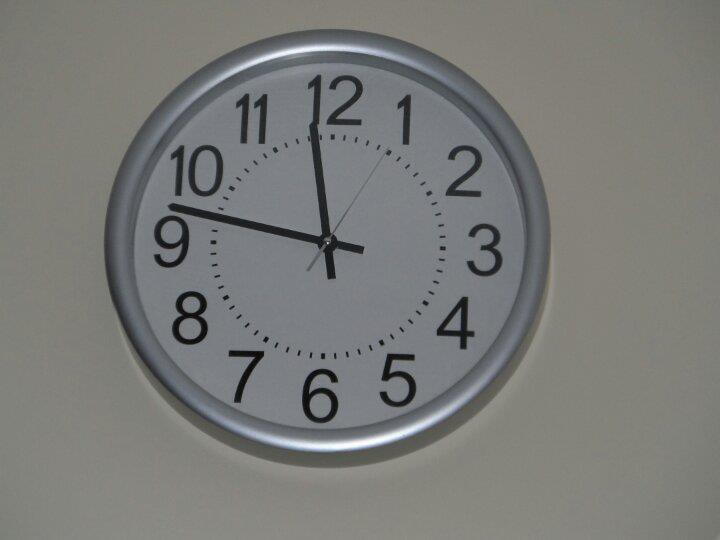A detailed colour photograph captures a round wall clock with a sleek silver frame. The lighting creates a reflective sheen on the top and bottom edges of the clock's rim, enhancing its polished appearance. The clock face is adorned with standard Arabic numerals from 1 to 12, embedded between distinct minute markers, with thicker lines signifying each hour. The black hour hand hovers just before the 12, while the black minute hand rests between the 9 and 10. A delicate, silvery second hand points precisely at the 1. The wall behind the clock has a subtle yellowish tint, and there is a faint shadow beneath the clock, suggesting that the primary light source is positioned above. The image is sparse, focusing solely on the intricacy of the timepiece against its plain backdrop.